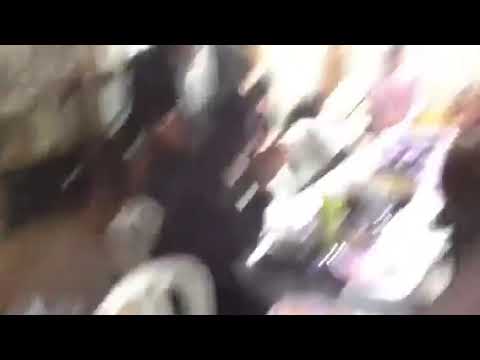The image is an extremely blurry and potentially accidental capture, characterized by significant motion blur and an overall lack of clarity. It features a man in a suit, identifiable by his dark attire and the suggestion of a black hat, although some details are obscured due to the blurriness. The man is illuminated by very bright lights, possibly indicating his proximity to a window or bright electronic light source, set against what appears to be an indoor wall. The image also includes black rectangular borders at both the top and bottom, framing the central chaotic blend of colors and shapes. In the upper right quadrant, there may be another faint figure or white shape, heavily distorted and difficult to discern clearly. The entire scene is enveloped in hues of pink, white, and dark areas, adding to the confusion and the impression of motion. The overall effect suggests a mishmash of shadows or light streaks, giving the appearance of an abstract painting rather than a traditional photograph.